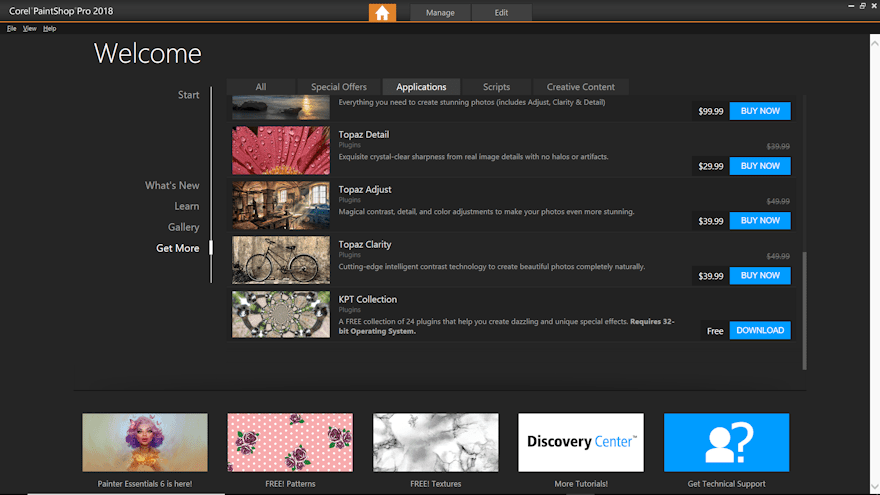The image depicts the interface of Corel PaintShop Pro 2018. At the top left corner, the title "Corel PaintShop Pro 2018" is displayed. Centrally placed at the top is a small house icon against a yellow background. To the right of the house icon, there are two buttons labeled "Manage" and "Edit."

Moving downwards, a series of categories are listed horizontally in the top middle section, including "All," "Special Offers," "Applications," "Scripts," and "Creative Content." The "Applications" category is currently selected, distinguished by its white text. To the left of these categories is the word "Start," with a vertical line extending downward from it. Below the "Start" label, four additional categories are listed: "What's New," "Learn," "Gallery," and "Get More."

At the very bottom of the image, five boxed areas span from the bottom left to the bottom right. The far-left box reads "Painter Essentials 6 is here." Moving right, the subsequent boxes are titled "Free Patterns," "Free Textures," "More Tutorials," and "Get Technical Support," respectively.